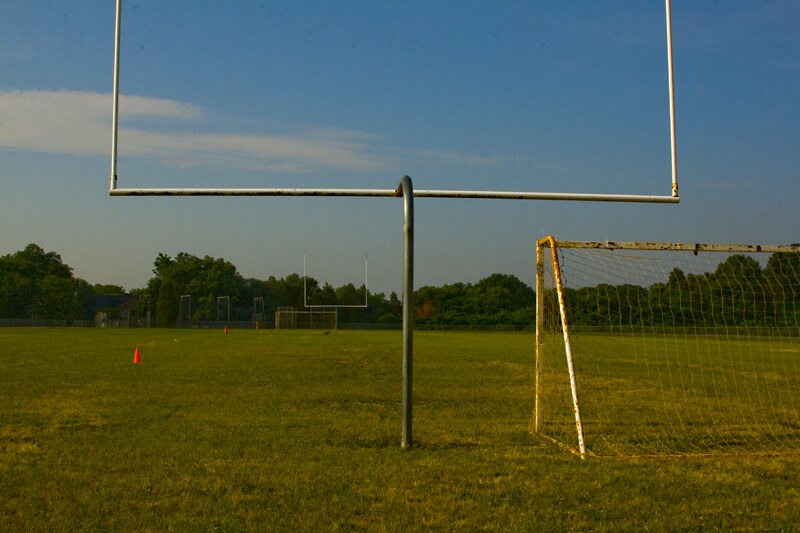This is an outdoor photo taken at a field that appears to be used for both soccer and football practice, captured just beyond a grass surface with patches of dirt. Dominating the foreground on the bottom right is a rusty soccer goal, and another one can be seen faintly in the distance behind the far football goal post. Spread across the field are several yellow and orange cones, likely used for marking practice areas. Prominently featured in the center, and mirrored on the opposite end, are large silver football goalposts. Surrounding the field is a fence, beyond which stands a line of lush green trees under a partially cloudy blue sky. The lighting suggests a time around dusk, casting a gentle, dimming light over the scene, adding a serene ambiance.